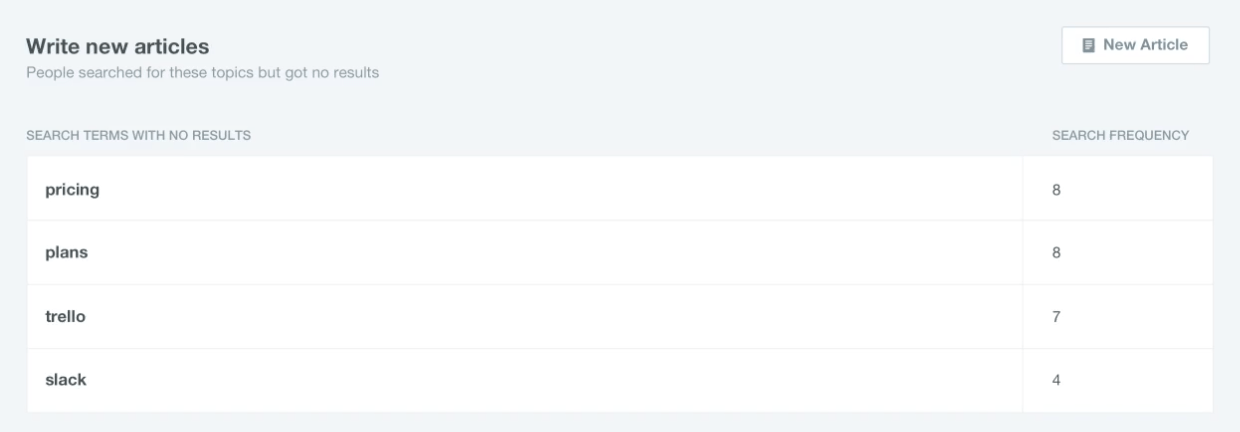The landing page is designed for users interested in writing news articles, likely catering to those involved in SEO management. The page sports a clean, minimalistic layout with a white background. Centered at the top, bold black letters headline the purpose of the page: "Write News Articles." 

Below this header, there is a section outlining search results for commonly queried topics, though it indicates that these search terms yielded no results. The specific search terms and their corresponding search frequencies are listed as follows: 
- "Pricing" with a search frequency of 8
- "Plans" with a search frequency of 8
- "Trello" with a search frequency of 7
- "Slack" with a search frequency of 4

On the upper right-hand side of the page, there's a prominently positioned button that invites users to create a "New Article." 

The entire layout, apart from the button, adheres to a monochromatic color scheme with black and gray text on a white backdrop, emphasizing simplicity and clarity. This streamlined design suggests it is tailored for users focused on search engine optimization (SEO) and content management, providing them with basic analytics and tools to track and generate articles efficiently.